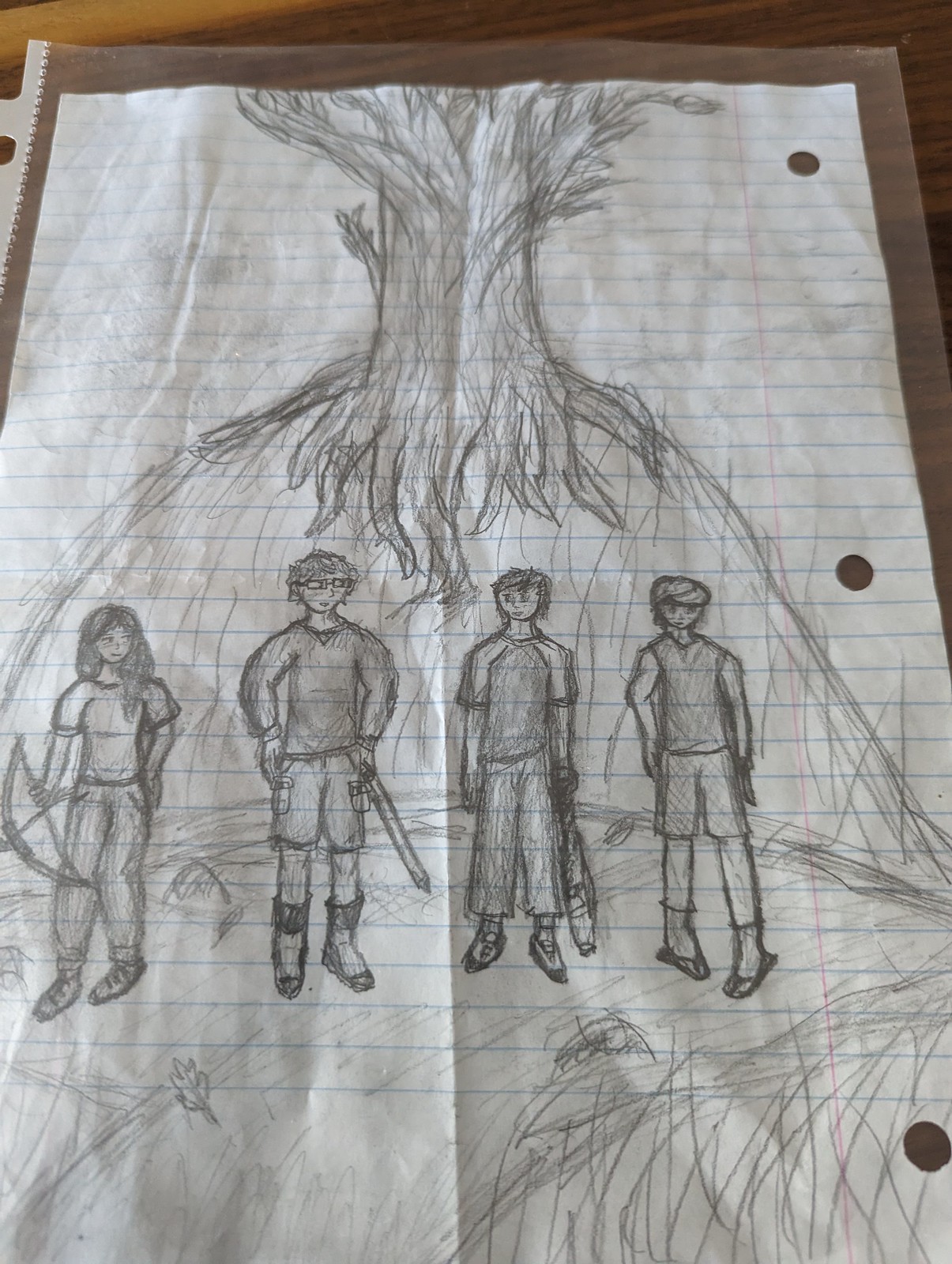A detailed pencil drawing on white lined notebook paper depicts a central tree atop a hill, its roots extending downward. The tree, only showing its trunk and roots, is surrounded at its base by four characters standing next to each other, each imbued with distinct details and expression. The scene appears to be protected in a plastic cover with the paper featuring three punch holes on the right-hand side.

Starting from the left, a young woman with long hair cascading over her shoulders and bangs is seen. She sports a short-sleeved shirt, jeans, and sneakers. With a smile on her face, she looks to the right, holding a bow with an arrow knocked in her right hand, while her left hand rests on her hip. Next to her stands a young man with shaggy short hair and square-framed glasses. He is also smiling and looking to the right, dressed in a long-sleeved shirt, shorts, and tall boots. A sword is visible, poking from behind his back.

The third character, another young male, is depicted with short hair and a smile directed at the person to his left. Dressed in a short-sleeved dark-colored shirt, long dark pants, and sneakers, he wields a baseball bat in his left hand. Lastly, the fourth individual with short hair is facing right, wearing a sleeveless top, shorts, socks, and sandals. Standing somewhat pigeon-toed, this character has their left hand by their side and their right hand on their hip. The characters are sketched in an amateur anime style, hinting that the drawing could have been created by a teenager.